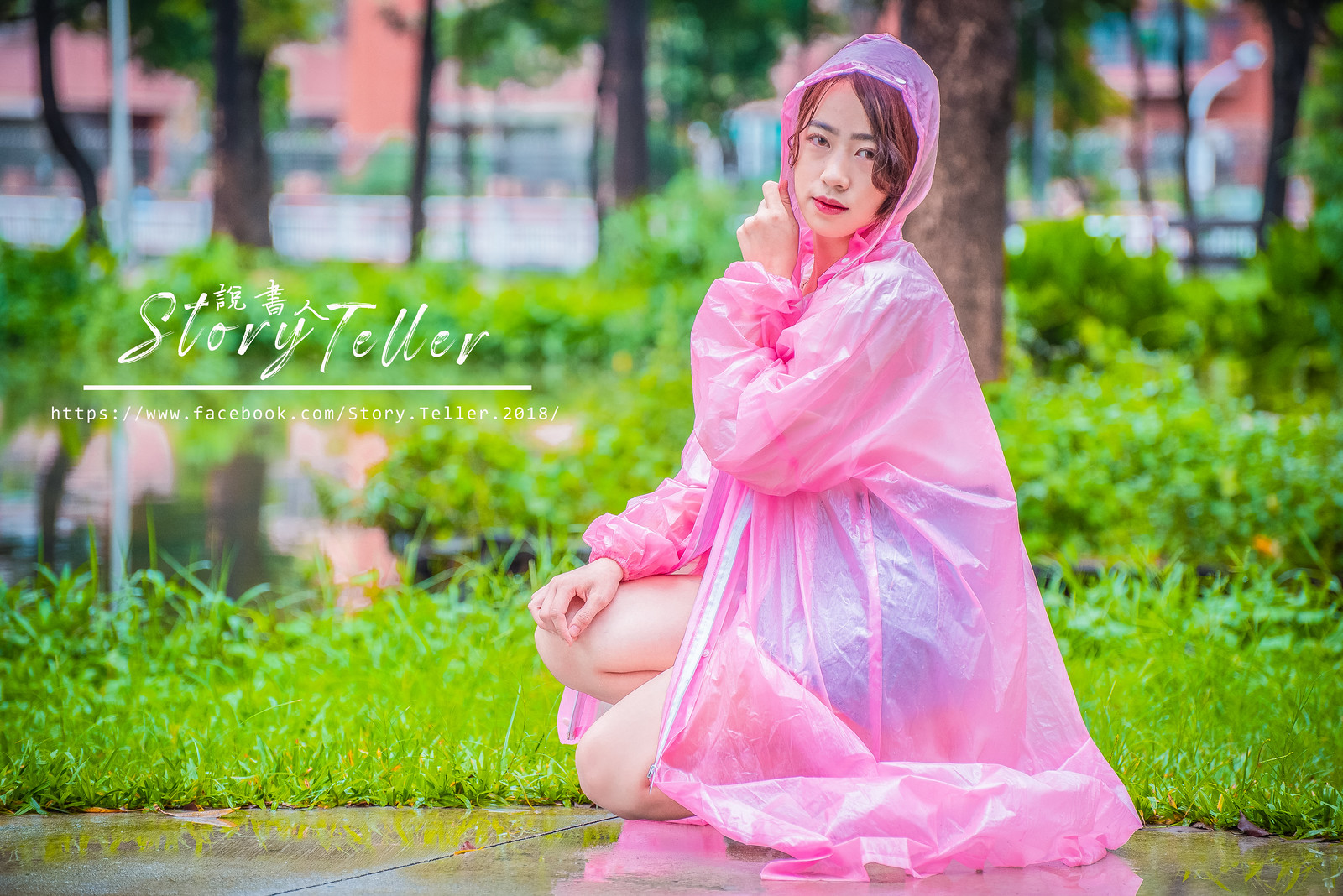The image depicts a young Asian woman with straight, dyed brownish-reddish hair, wearing pink lipstick. She is dressed in a translucent pink raincoat with a hood, which is partially covering her head, and shorts. She is kneeling on a wet sidewalk, facing to the left with her head turned towards the viewer. Behind her is lush greenery, including green grass, low shrubbery, and some trees, likely indicating a city park as buildings are faintly visible beyond the trees. Her expression is neutral. Superimposed on the image, in white handwritten type font, is the word "Storyteller," along with a URL: "https://www.facebook.com/story.teller.2018/".